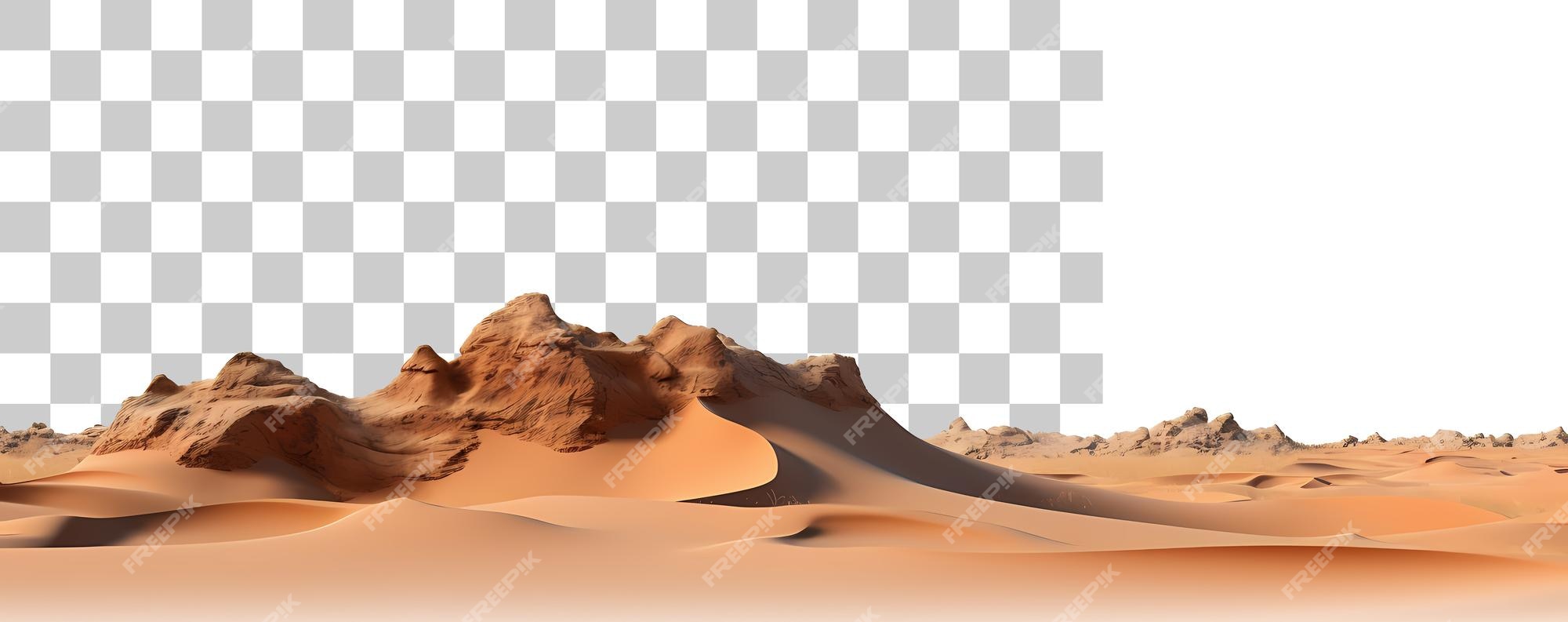This image portrays a desert landscape with light tan sand dunes encompassing rocky formations, whose slightly darker brown hues contrast subtly with the surrounding sand. The dunes are primarily situated around these rocky outcrops and exhibit gentle curves, creating a dynamic, undulating terrain rather than flat expanses. Toward the left of the image, the background features a checkerboard pattern of gray and white, while the right side transitions to a solid white backdrop, suggesting parts meant for transparency. In the distance on the right, smaller rocky hills are visible. The image is overlaid with a watermark that reads "Freepik," and this overlay covers significant portions of the scene, including areas of visual interest.